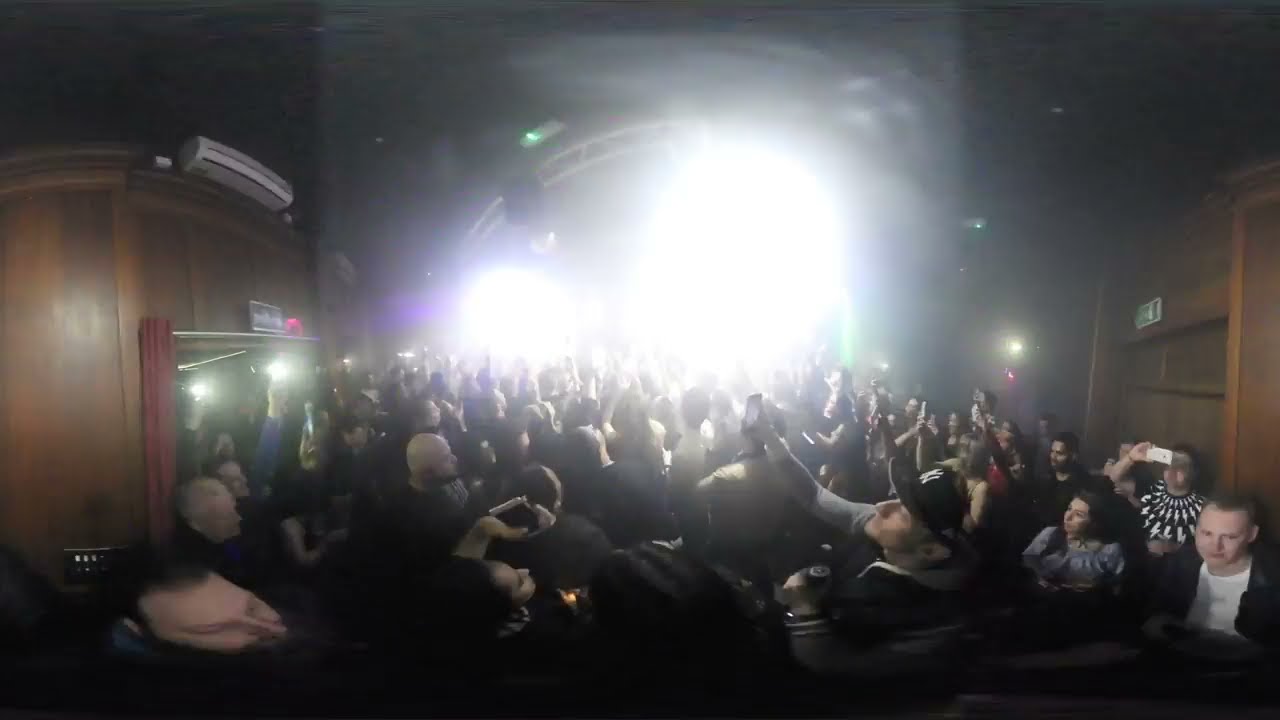This image captures a wide-angle shot of a bustling indoor dance club, shrouded in darkness but illuminated by vibrant lights. Centrally, a large crowd of people huddles closely together, many holding up their cell phones to capture photos and videos of the performance on stage. The stage, situated at the far back, is faintly visible under the glow of purple, green, and yellow lights emanating from the ceiling and a smoke machine that casts an ethereal haze. A DJ stands behind a microphone, framed by a round gong, while a disco ball hangs high above, adding to the club's energetic ambiance. The venue appears narrow and elongated, with wooden walls on the left and right sides, and possibly a couple of bars flanking the crowd. The overall setting suggests a lively night-time event, filled with a diverse mix of colors—black, brown, white, pink, purple, gray, yellow, and tan—capturing the dynamic atmosphere of this crowded club.